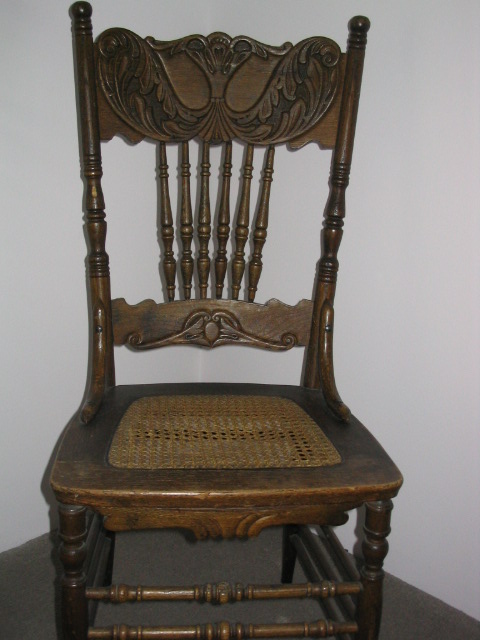This image showcases an intricately carved antique wooden chair positioned in the corner of a room with white walls and a dark floor. The chair, likely dating back to the early 19th century or earlier, features a high back adorned with detailed engravings resembling ocean waves. The backrest is supported by six spindles connecting the top and lower sections. The chair's sides are flanked by tall uprights with old-fashioned curved braces that attach to each rail and the seat. The seat itself is made of cane embedded in wood, with a hole that has been covered with a softer material for comfort. The chair's lower horizontal section also includes fine carvings and has spindles—two running between the front legs and three connecting the front to the back—to provide additional stability. The setting appears to be indoors, and there are no other objects in the photo, emphasizing the chair’s central prominence against the simple white walls and dark flooring.